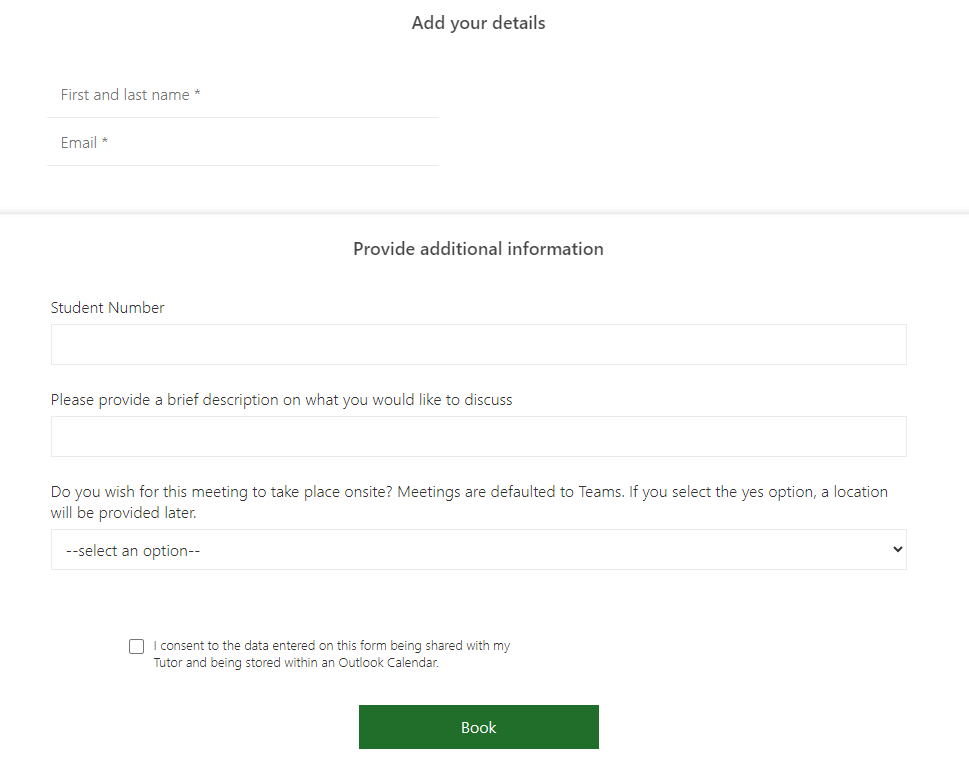The caption submitted appears to have been transcribed with unnecessary instructional text. Here's a cleaned-up and detailed descriptive caption based on the provided elements:

---

"In this image, a green book is prominently placed in the foreground. Behind the book, a button can be seen, adding a subtle yet intriguing depth to the scene. The green book’s cover is textured and reflects a soft ambient light, while the button, partially obscured, hints at an underlying story waiting to be discovered."

---

For clarity, all unrelated content has been omitted from the original poorly transcribed request.